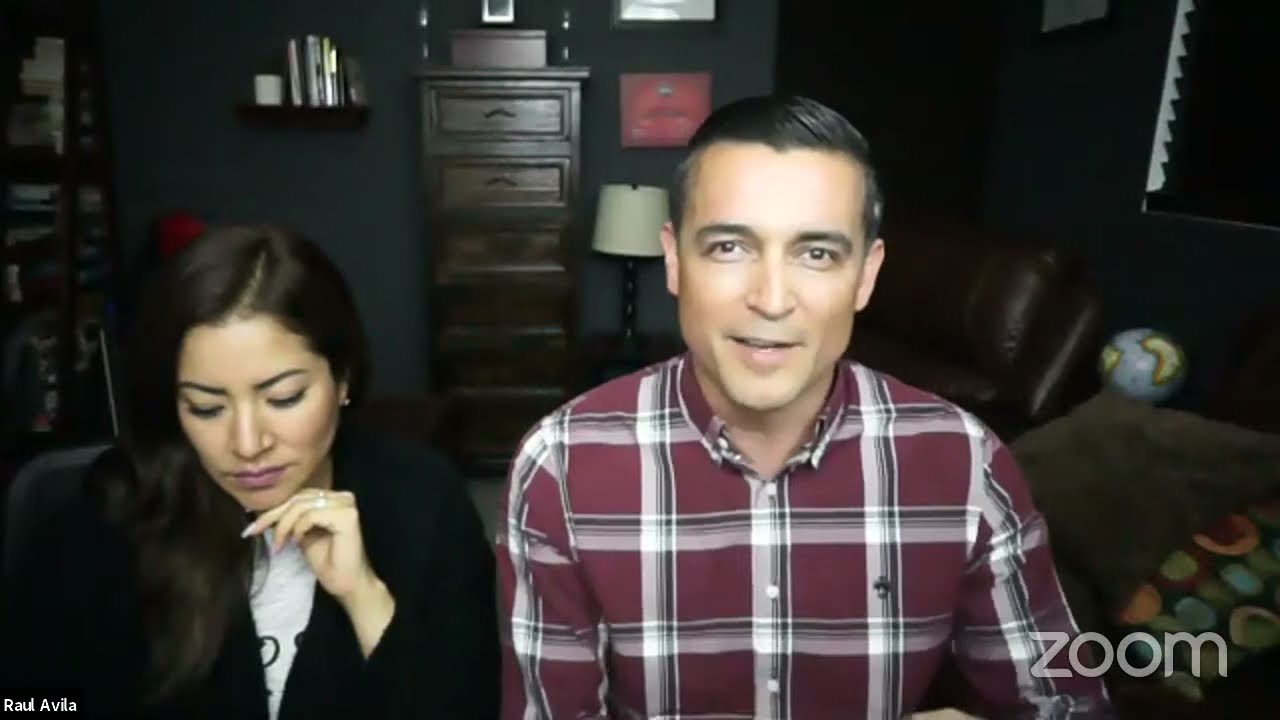In the image, a screenshot of a Zoom meeting, there are two people prominently displayed, with the Zoom logo in gray text at the bottom right corner and the name "Raul Avila" in white text at the bottom left corner. Centrally positioned is a man in his early 50s with brown skin, neatly trimmed dark brown hair that has specks of gray. He is wearing a plaid shirt with maroon, red, and white stripes. To his left, a woman in her early to mid-40s with long dark brown hair wears a black jacket over a white shirt. She appears to be looking down, possibly at her phone, and is resting her chin on her hand, which has rings on it.

They are seated in a room with a tealish-green wall. In the background, there is notable furniture including a tall brown dresser, a dark black lamp with a white shade, and a brown chair or couch adjacent to the lamp. A window with blinds is situated at the very top right of the image, beneath which is a blue globe with green continents. The general setting suggests a moderately busy living room, decorated with various everyday items including a bookshelf mounted on the wall that holds books and a small candle.